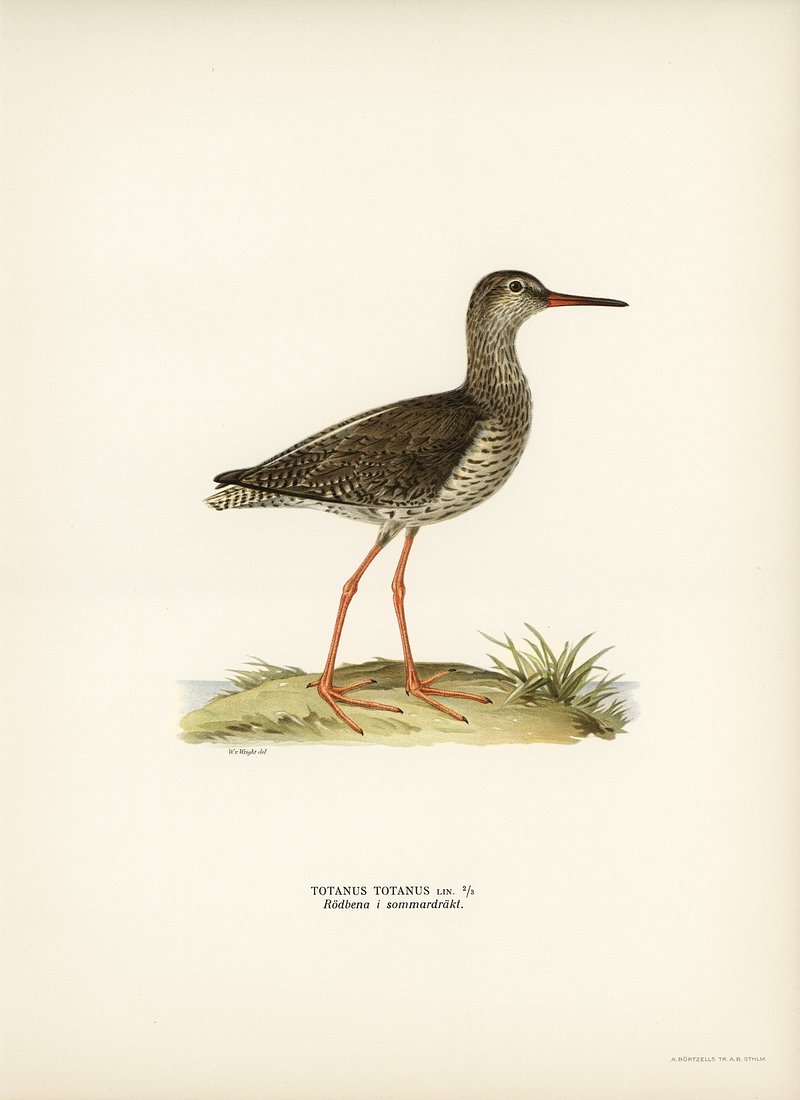The image captures a Totanus totanus bird, distinguished by its long, slender, orange legs and sharp, extended beak. The bird features a medium build with brown and white feathers, with the chest displaying a lighter, grayish hue adorned with small spots. Its wings are dark brown, accented by white tips, and it has a small, rounded head. The bird stands atop a grassy mound, surrounded by hints of green plants and barely visible water on either side, suggesting a coastal setting. The bird appears to be in a moment of alert observation, set against a natural landscape. An artist’s faint signature is visible beneath the mound, completing the serene scene.